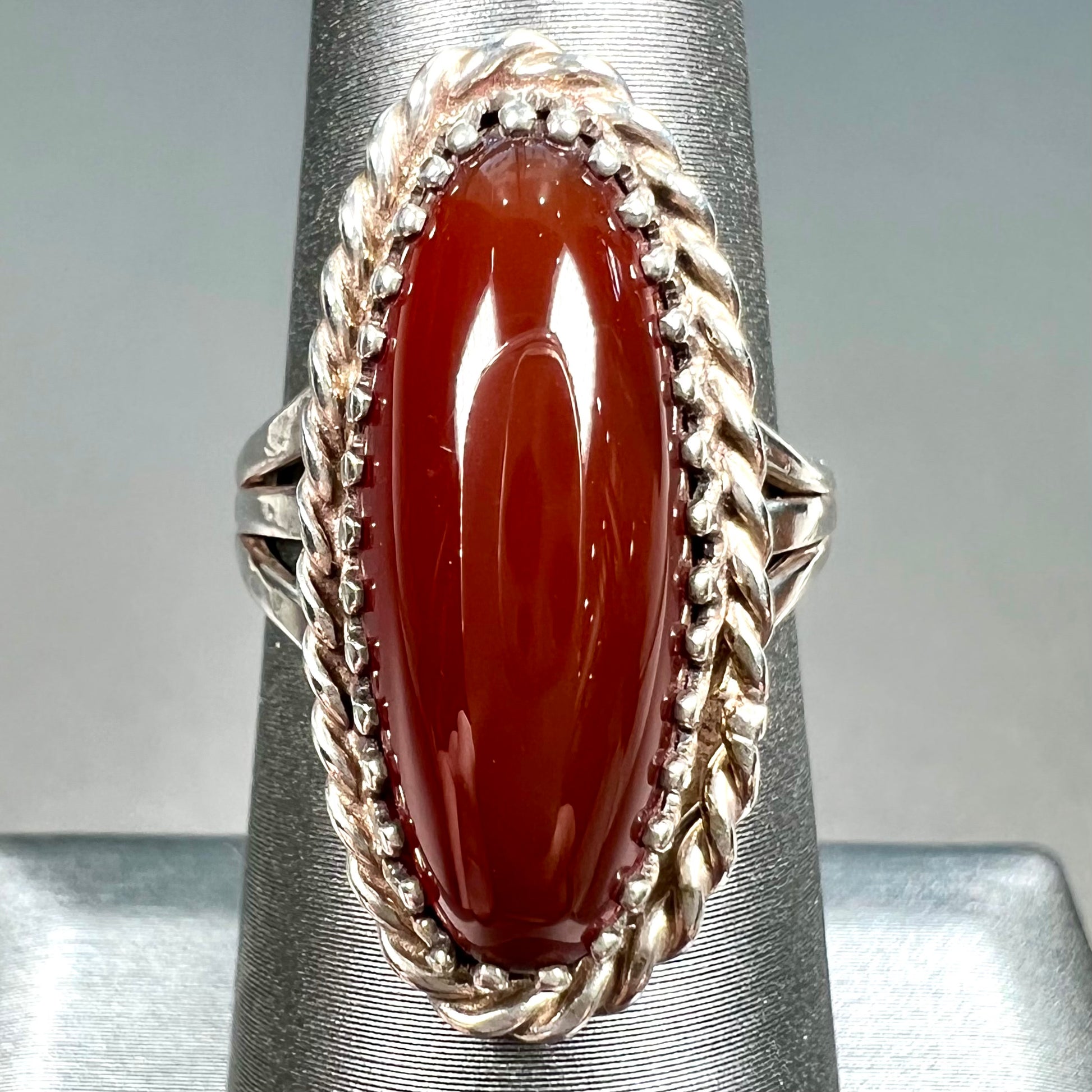The image is an extreme close-up digital photograph of a striking jewelry ring, with a richly detailed focus on its various elements. At the center of the image is a large, silvery ring elegantly propped upright on a silver cylinder, simulating a finger wearing it. Dominating the scene is an oblong, oval-shaped gem set within the ring. This gem is an opaque, deep red color, notable for its large size and its shiny, smooth surface that makes it appear glossy and polished. 

Encircling this grand central stone is a decorative ring of small, glittering diamonds, adding to the luxurious appeal of the piece. The band of the ring is also silvery and features intricate silver swirling patterns that enhance its ornate design. The ring's setting gives off both silver and bronze hues, creating a rich visual contrast against the gem. The background reveals that the ring and its stand rest on a silver table, with a muted gray wall serving as a backdrop, further directing attention to the stunning jewelry centerpiece.